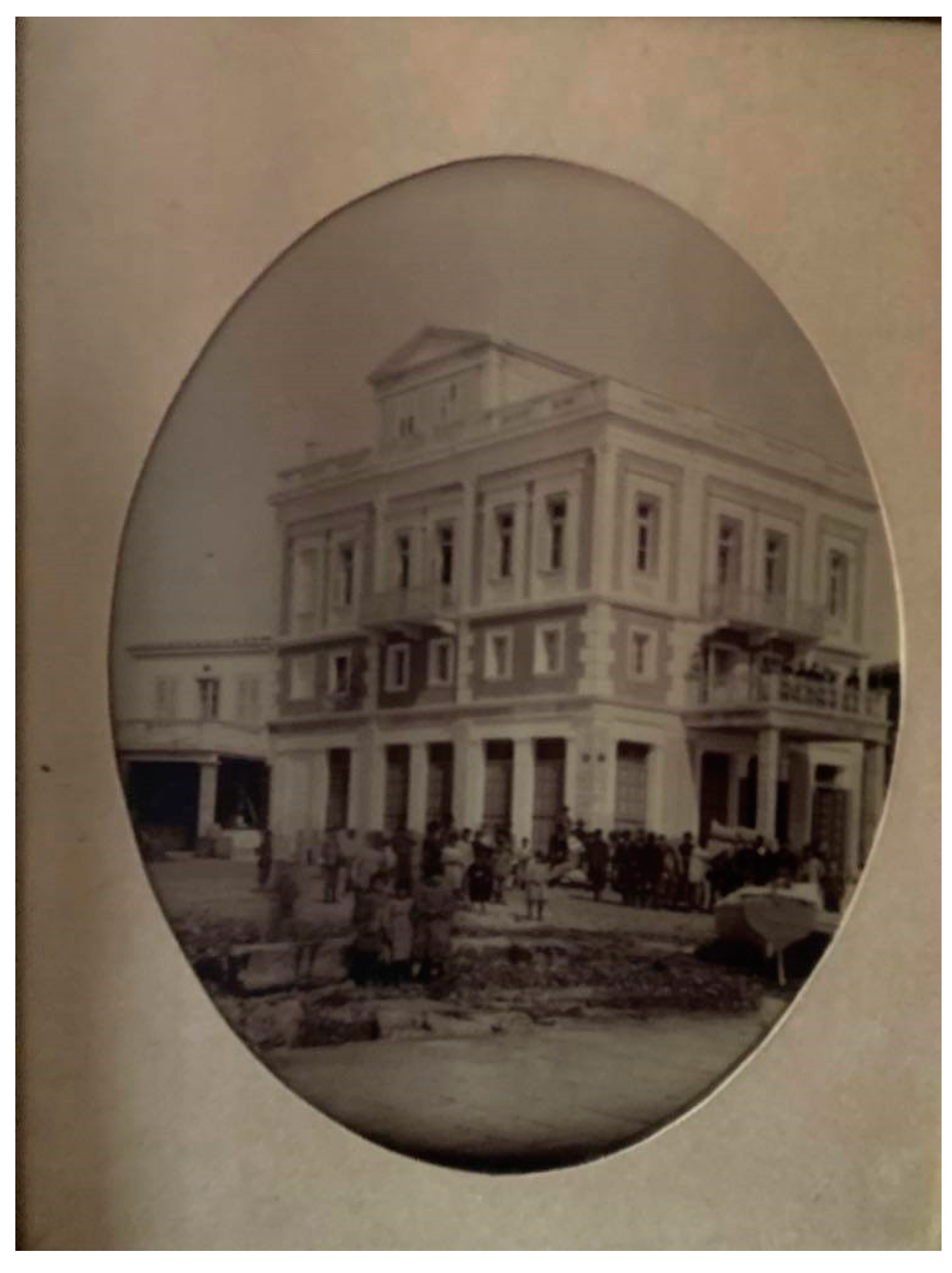The black and white, oval-shaped image fixed on a white surface depicts an old-fashioned, three-story white building with numerous windows and doors. The front of the building is prominently on the right side of the image, featuring an entrance flanked by two pylons and surmounted by a balcony where people are standing. The ground floor is bustling with many individuals dressed in vintage outfits suggestive of the 1950s, 60s, or an even earlier era. The image also shows a second balcony to the left with additional pillars underneath. Although the details are somewhat obscured in the black-and-white format, the ground appears possibly muddy. The overall scene captures a historical moment with a crowd gathered around the building's exterior.